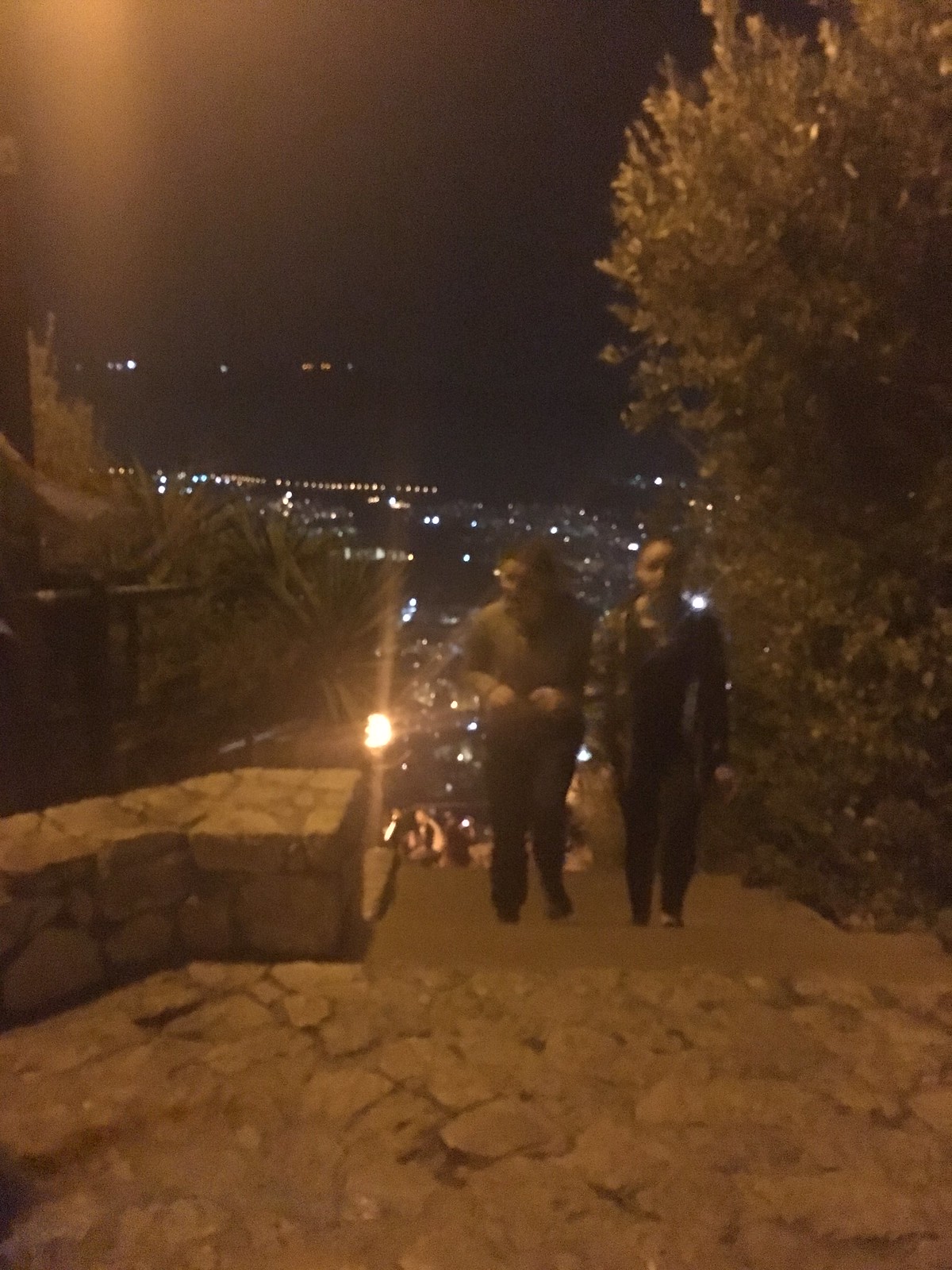This blurry nighttime photo captures an outdoor setting, possibly in a warmer climate, filled with vibrant city lights in the distance. The image is taken from an elevated cobblestone area, looking down on a wide set of cement or stone stairs. These stairs are framed by lush trees and mature bushes on both sides, with fronds visible on the left and dense leaves or a tall bush on the right. Two people in long sleeves and long pants, appearing to be young, walk up the stairs, seemingly focused on the camera. Behind them, several more individuals are ascending, adding to the sense of a lively, albeit blurred, night scene. The completely black sky accentuates the distant city lights, creating a striking backdrop for this bustling urban tableau.